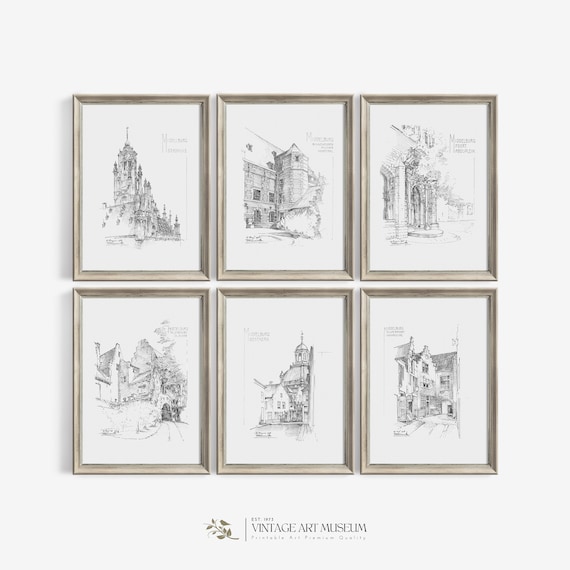This image showcases six detailed pencil sketches of historical buildings, each framed in weathered white wood. The artworks are set against a white background. The top left sketch features a castle with numerous pointed turrets. The top middle drawing depicts a castle with a single prominent spire. The top right illustration shows an architectural walkway framed by pillars. The bottom left artwork includes houses and trees, suggesting a quaint residential area. The bottom middle sketch appears to be of a church, distinguished by its significant spires. The bottom right image resembles an alleyway leading to a store. Beneath the framed drawings, there is a logo reading "Vintage Art Museum" with some partially obscured text.